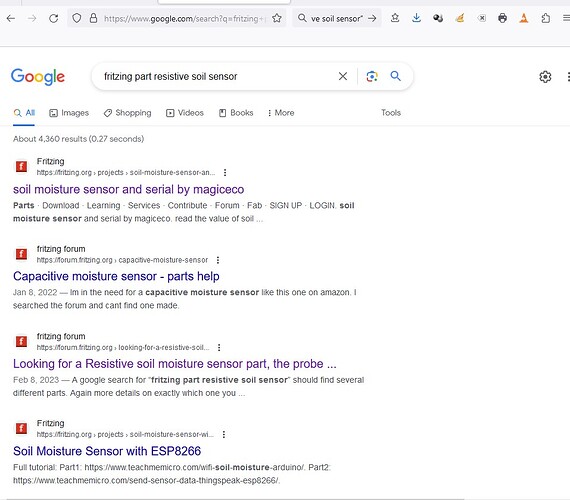### Detailed Caption for Screenshot of Google Search Results:

The screenshot captures a Google search results page. Across the top section from left to right, key browser navigation icons are visible: a back arrow, a forward arrow, a refresh button, and a shield symbol with a lock, indicating a secure connection. The address bar displays "google.com" with an active search for "Fritzing Part Resistive Soil Sensor." Adjacent to the address bar are a bookmarks button, an additional search bar, another bookmarks-related button, downloads, and several icons with distinct appearances, including a bomb, a sailboat, a delete button, a printer, a safety traffic cone, and a puzzle piece. On the far right, three vertical black lines provide access to the browser menu.

Below the navigation bar, the Google logo is located on the left, adjacent to the search input box containing "Fritzing Part Resistive Soil Sensor." To the upper right of the search results area are settings gear and three vertical dots opening another menu.

The primary search results are displayed below, predominantly sourced from "fritzing.org." The first result, tagged "Soil Moisture Sensor and Serial by Magic Eco," includes a description focusing on reading soil moisture values. The second result, "Capacitive Moisture Sensor Parts and Help," features a forum post discussing the need for a capacitive moisture sensor and how to locate one on Amazon. The third result, "Looking for a Resistive Soil Moisture Sensor Part at the Probe," provides guidance on finding different parts related to the search query. The description includes the text "a Google search for Fritzing Part Resistive Soil Sensor should find several different parts," offering advice on locating specific components. Finally, a fourth result titled "Soil Moisture Sensor with ESP8266" includes a tutorial link, detailing part 1 and part 2 instructions for utilizing the soil moisture sensor.

The screenshot highlights a neat and organized presentation of technical resources from Fritzing's official site and its forum, aimed at assisting users in locating soil moisture sensor parts and related information.